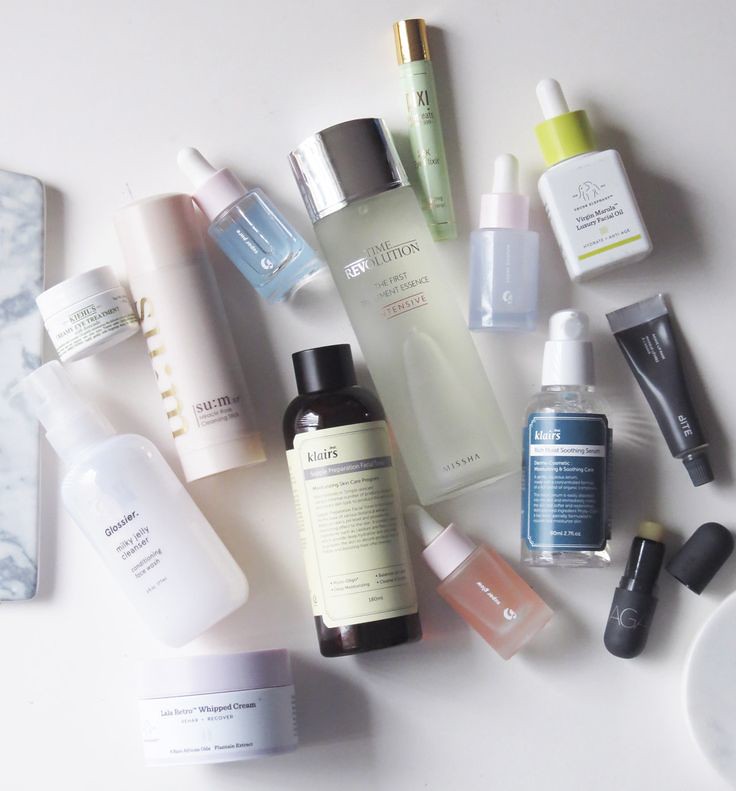The image showcases an array of various skincare products, seemingly from a recent skincare haul. The items are meticulously arranged on a white surface, which could be a table, vanity, or bathroom countertop, creating a clean and minimalistic backdrop. The collection includes bottles and tubes from different brands, each with distinctive packaging.

The most prominent item is a sheer glass bottle labeled "Time Revolution," filled with a clear liquid and topped with a sleek silver cap, exuding sophistication and elegance. Next, a black tube of chapstick is noticeable, with its cap removed and the clear, no-color balm twisted up, ready for use. Additionally, a transparent bottle of Glossier Milky Jelly Cleanser stands out, equipped with a nozzle for convenient application. Adding a unique touch to the assortment is what appears to be a facial whipped cream, although the specific details of this product are less discernible. This diverse collection, carefully displayed, highlights a well-rounded skincare regimen shared for social media admiration.